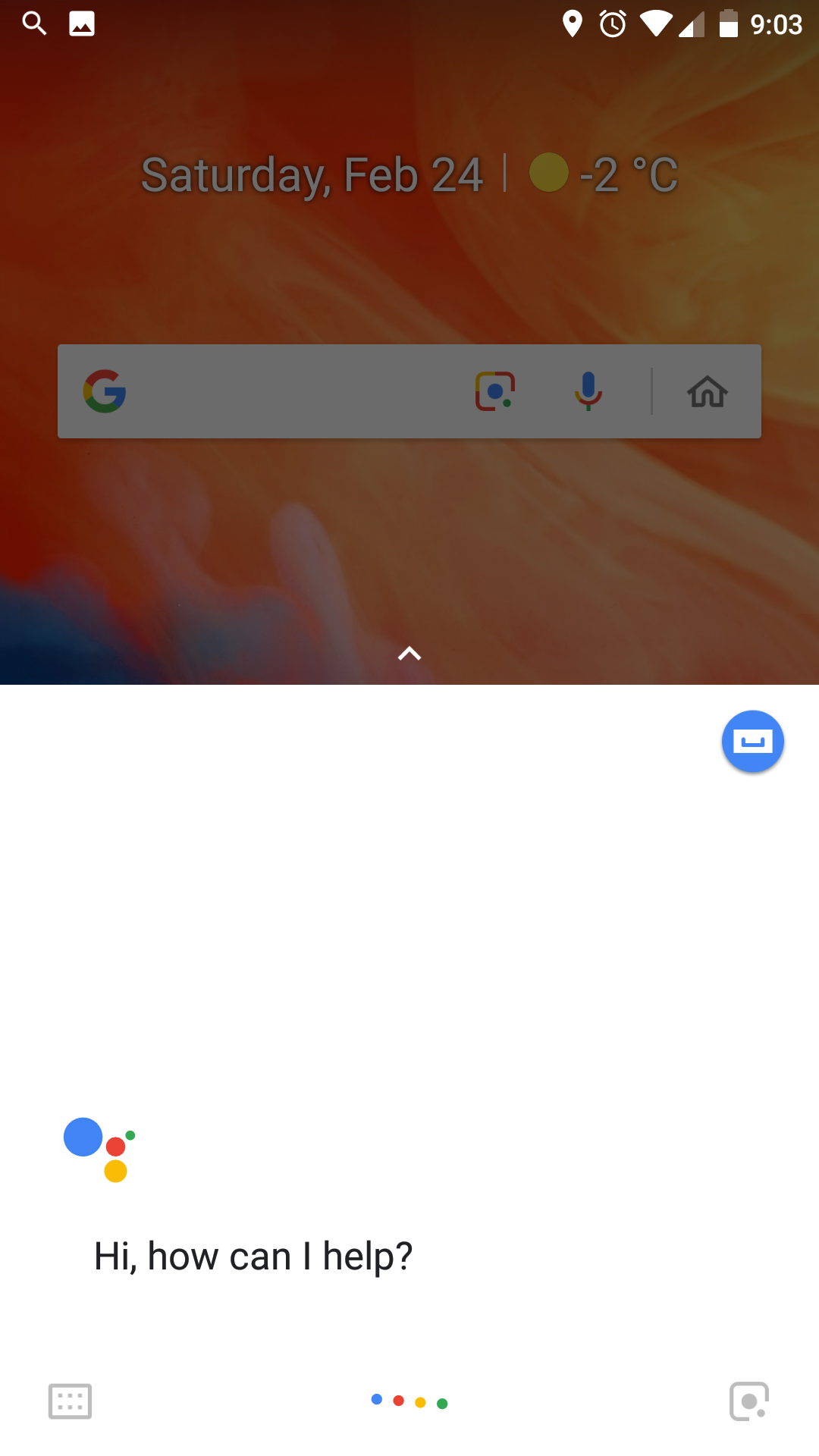This image showcases a cell phone screen with various interface elements. At the very top left, there is a search bar icon followed by a gallery icon. On the top right, there is a clock displaying the time as 9:03, alongside Wi-Fi, connection, and battery percentage icons. Just below these indicators, though faded and dim, the text reads "Saturday, February 24th, -2°C".

Centered below this information, there is a Google search rectangle featuring a "G" lens icon on the left, a microphone icon in the middle, and a home icon on the right. The background behind this search bar is predominantly orange, with slight touches of yellow and blue.

Beneath the Google search bar, a blue circle with an email icon can be seen. At the very bottom, a text prompt states, "Hi, how can I help?" This is part of a Google chat feature.

The lower half of the screen displays a white background. On the bottom left, there is a keyboard icon next to a Google logo represented by a blue dot, red dot, yellow dot, and green dot. On the bottom right, there is a camera lens icon.